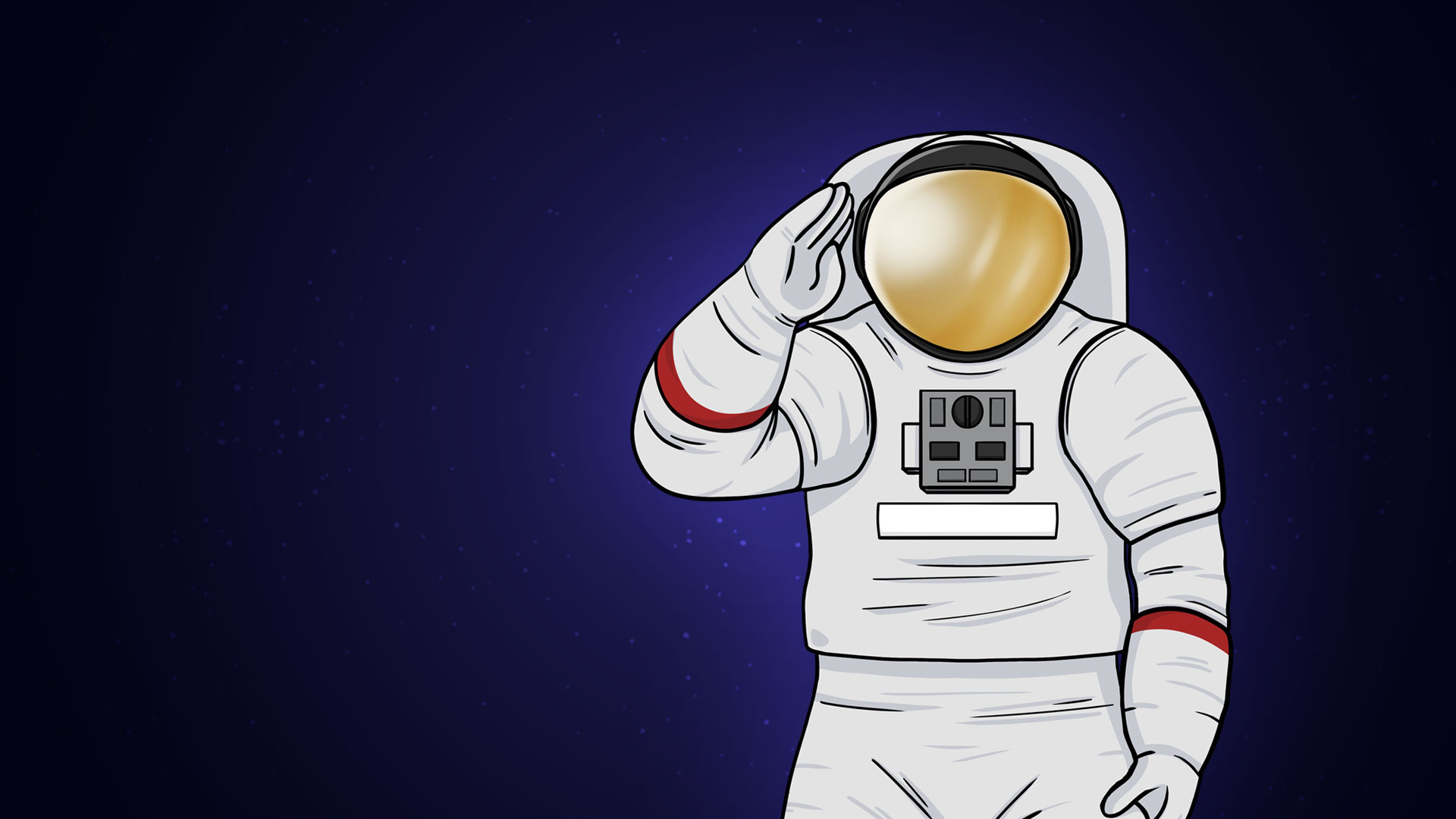The image is a detailed, cartoon-style drawing of an astronaut set against a softly transitioning background that fades from a very dark blue on the left to a rich royal blue on the right. This background includes the faint outline of stars, enhancing the feeling of a deep-space environment. The astronaut is depicted in a clean white suit, featuring a couple of striking red rings around both forearms just beneath the elbows. The front of the suit showcases a gray box equipped with several buttons, likely part of the control panel, and a white stripe or bar situated underneath it. The astronaut's head is adorned with a black helmet that sports a reflective, gold visor, concealing the face entirely. Further adding to the astronaut's gear is a white backpack visible on the back of the suit. The limbs of the astronaut appear padded, giving them a bulkier appearance, and a pair of thick gloves are noticeable. The stance of the astronaut is one of salute, with their right hand raised in this gesture. The overall artwork is enclosed in a rectangular frame, contributing to its orderly presentation and clear focus on the spacewalking figure.